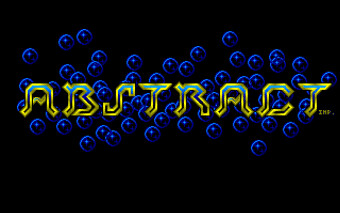The image showcases a pixel art title screen from a video game, reminiscent of classic Sega Genesis or Master System aesthetics. Dominated by the word "abstract" in the center, the text features a blue-to-black gradient with a yellow-to-gold outline as it reaches the top. The unique, stylized font includes tiny letters "IND" to the right of "abstract." The background is a solid black adorned with blue-outlined bubbles that have reflective highlights, adding depth and a light source effect. The compact size of the screenshot enhances its retro, low-resolution charm.